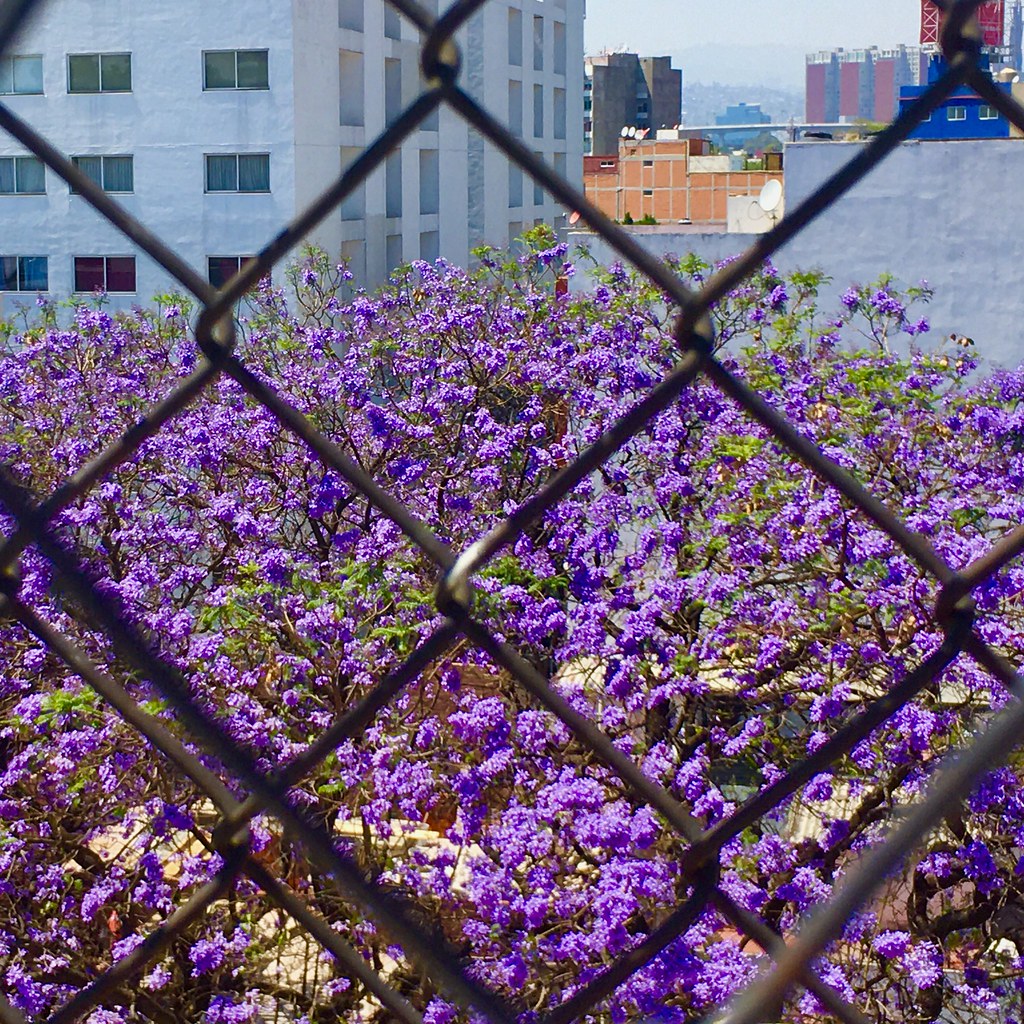This image is a detailed daytime photograph taken outdoors, framed within a six-by-six-inch square. Dominating the foreground is a silver chain-link fence, its diamond pattern distinctly visible. Beyond the fence, a large bush with vibrant clusters of purple flowers spans the bottom two-thirds of the image. Amid the profusion of blooms, patches of green leaves and budding flowers are interspersed. In the upper portion of the image, a considerable stone building with at least four stories and closed windows stands prominently on the left-hand side. The right side reveals a bustling city skyline with an array of tall buildings, including an orange brick structure, a blue building, a pink and blue edifice, and a brownish-gray one. The backdrop is capped by a somewhat hazy blue sky, indicative of a typical smoggy urban environment.